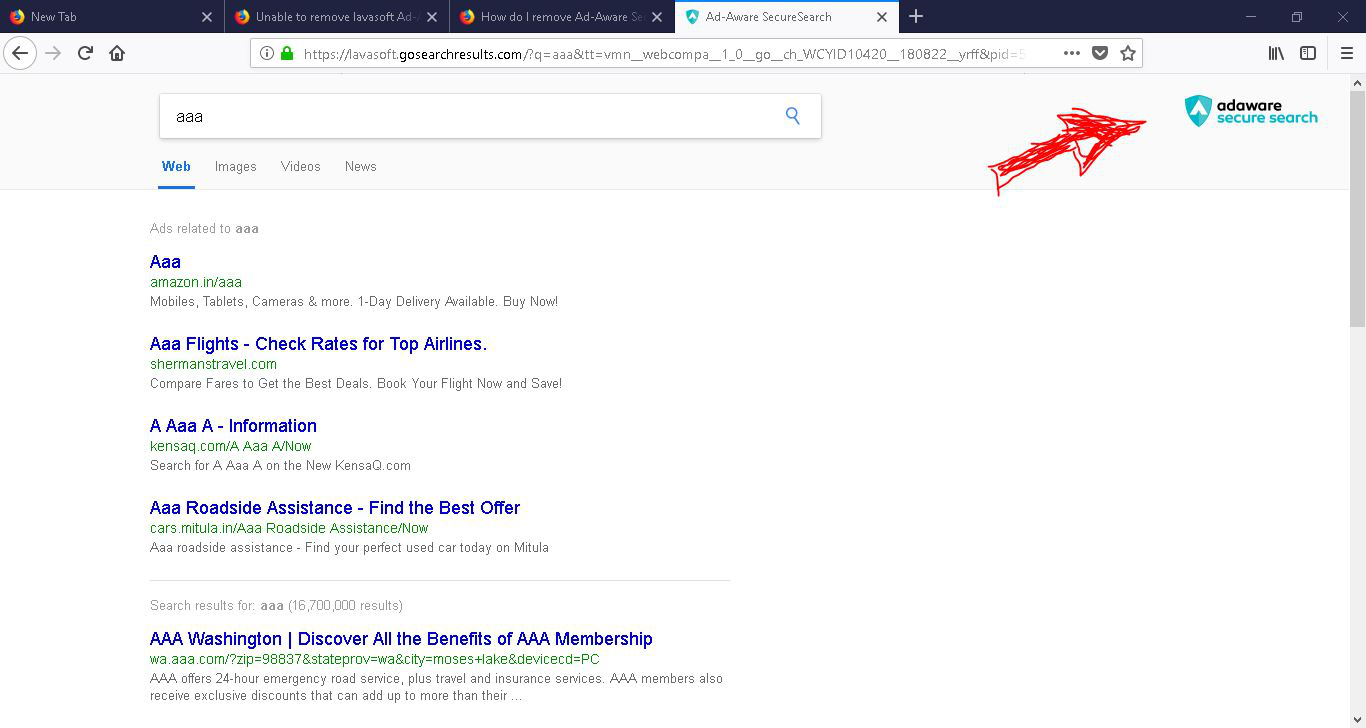At the very top of the page is a long black rectangle. Below this, there is a white-highlighted area featuring the options: "Add," "Archive," "Save," and "Secure Search." To the side of these options, there is a blue upside-down triangle with the letter "A" inside. Directly underneath, an open search bar displays three lowercase "a's."

Beneath the search bar are navigation options labeled: "Web," "Images," "Videos," and "News." Additionally, there is a drawn arrow pointing towards a section labeled "Adaware Secure Search," which contains another upside-down triangle, this one in a bluish-green shade with an "A" inside.

Within the search bar area, pre-filled search suggestions related to the entered "aaa" include: "AAA's," "Amazon-AAA," "AAA Flights," "AAA Information," "AAA Roadside Assistance," "Find the Best Offer," and "AAA Washington" with the subtext "Discover All the Benefits of AAA Membership." All of these suggestions are displayed in blue text.